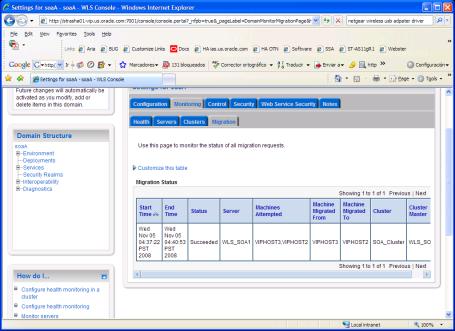**Detailed Caption for Screenshot of Windows Internet Explorer Settings Page:**

This image is a screenshot of the settings interface for Windows Internet Explorer. The iconic blue and white arrow pointing left, encased in a blue circle, signifies the browser's back button. Adjacent to it is a grey arrow pointing right, representing the forward navigation button. The address bar contains a partially legible web address starting with "HTTPS." The address appears to be something like "lupusitgrade.com," but the text is blurred and difficult to read.

Below the address bar, there are standard browser menu options, including "Edit," "View," "Favorites," "Tools," and "Help." Above these menus, a green-highlighted top line displays various links with labels such as "E for Ara," "D for Dario," "C for Customer Links," and others labeled as "Docs," "5-something," "6 PAC," "7 Software," "8 SGA," and "9 ET."

Further down, another line of text includes terms that are somewhat unclear due to the blurriness of the image. Phrases like "Mercadones," "connector strengths," "connector infograph," "logistics," and possibly "art logistics" are partially visible.

On the right side of the image, there is a grey vertical bar featuring a blue rectangle with the phrase "Settings for SAM4" or possibly "for Canada." The interface includes a home button and a print button situated on the top-right corner.

To the left side, there appears to be a menu board, but the top part is cut off. The visible text mentions "future terms will automatically link D1" and some references to "the mouse" and "2008."

Further elements of the interface list terms such as "environment," "checkouts," "services," "security," "rewards," "horoscope," "daily," and "sciatostica." Below these, additional terms seem to mention "kegs, casts, tests" and "medicine, test servers."

On the right side of the screen, a column is segmented into tabs with titles such as "configuration," "security," "food service secretary," and possibly "mad mayor" and "casserole." Below this, the page content states: "Use this page to meet the status of all migration requests," followed by customizable table headers including "Migration Status," "Start Time," and specific details like "November 5th, 4:37.22 PST."

In the table data, there's a list detailing migration progress with entries like "server wls 9041," "5041 on me," and specifics about machine statuses, such as "interrupted" and "inactive." Migration activities are detailed, like "machine be graded from wp host two" and "inactive, not to migrate to p host."

The image overall reflects the technical and somewhat cluttered layout often associated with Internet Explorer's settings and administrative interfaces.